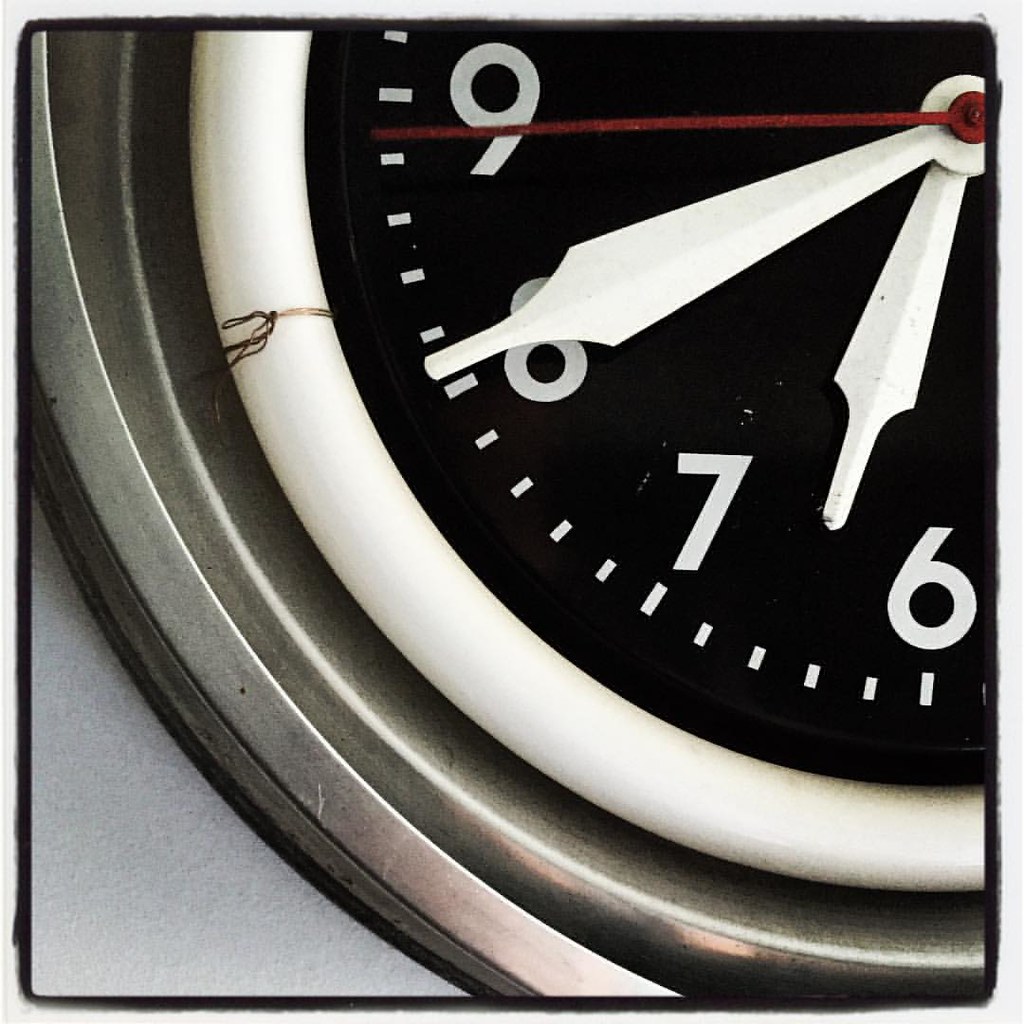This captivating image predominantly showcases a detailed close-up of a clock, which occupies the majority of the frame. The clock features a sleek silver outer rim, followed by a narrow white band encircling its central black face. Noticeably, the left side of the white band has a small string delicately tied above the number 8, about one minute past it. The black face prominently displays the numbers 9, 8, 7, and 6, with intricate white markings providing a stark contrast. The clock is equipped with two white hands: a large one just past the number 8 and a smaller one slightly beyond the number 6. A vibrant red second hand stands out against the monochrome elements. In the lower left-hand corner, a sliver of gray subtly appears, however, the clock commands the viewer's attention as the focal point of the image.